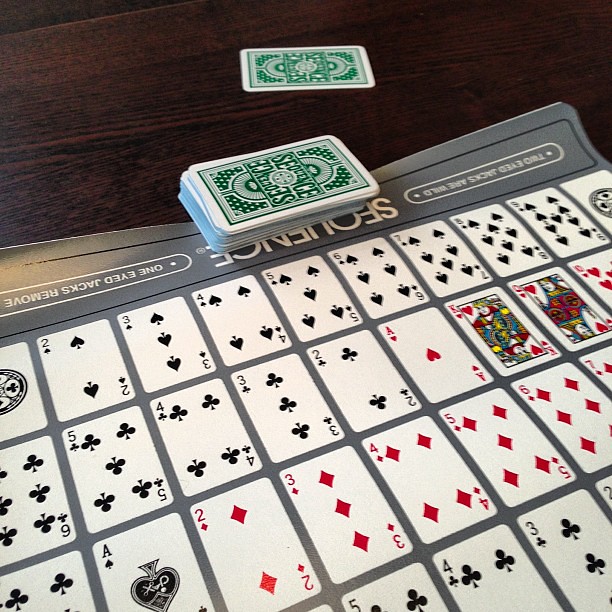A detailed photograph captures a rolled-up poster that has been flattened out on a dark, almost black wooden table. The poster prominently features the word "Sequence" along its border and displays an array of playing cards meticulously arranged. The visible portion highlights cards from the spades suit, specifically from 2 to 9, although the entire image is not shown. The poster seems to explain the rules of a card game named Sequence. Notably, it includes information about the rule variations for Jacks: one-eyed Jacks can remove a card, while two-eyed Jacks are considered wild. The poster is being held open by a stack of playing cards, with one card lying separately on the table beside the stack.